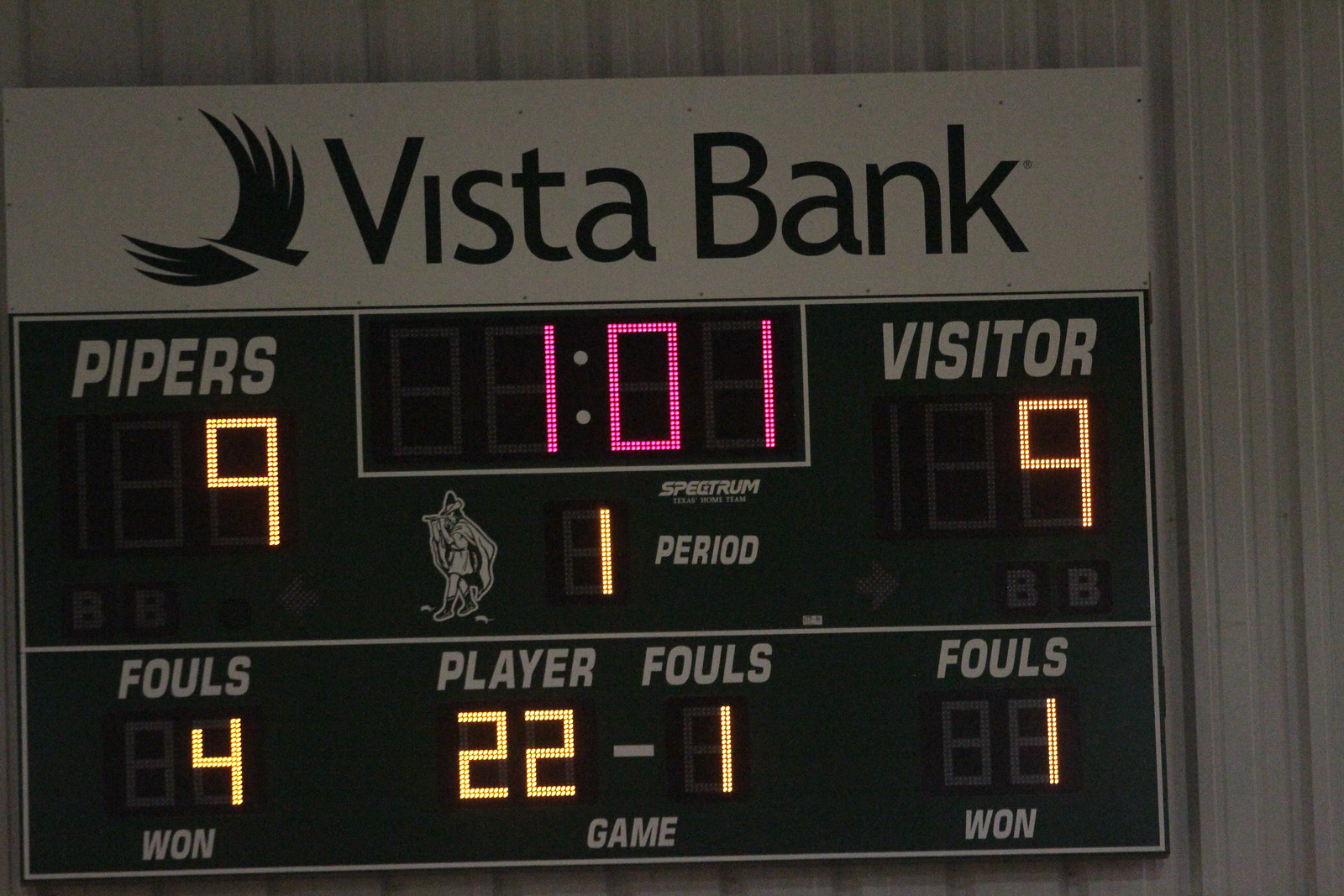This color photograph captures a close-up of an electronic scoreboard mounted on a corrugated metal wall. At the top of the scoreboard, the text "Vista Bank" is prominently displayed, indicating the sponsor. Adjacent to this text is an emblem featuring a large bird, possibly an eagle or another bird of prey, with its wings spread wide. The scoreboard’s primary display reveals that the home team, the Pipers, and the Visitors are tied with scores of 9 each in the first period. The time remaining is shown in pink numerals, with 1 minute and 1 second left on the clock. 

The scoreboard further details various fouls: the Pipers have committed 4 team fouls, whereas the Visitors have 1. In the middle section, it is noted that player number 22 has committed 1 foul. The text and numbers, except for the time, are illuminated in yellow, while the overall structure of the scoreboard features a green backdrop. Additionally, there is an image of the Pipers' mascot, depicted as an old man playing a pipe, reinforcing the team’s identity.